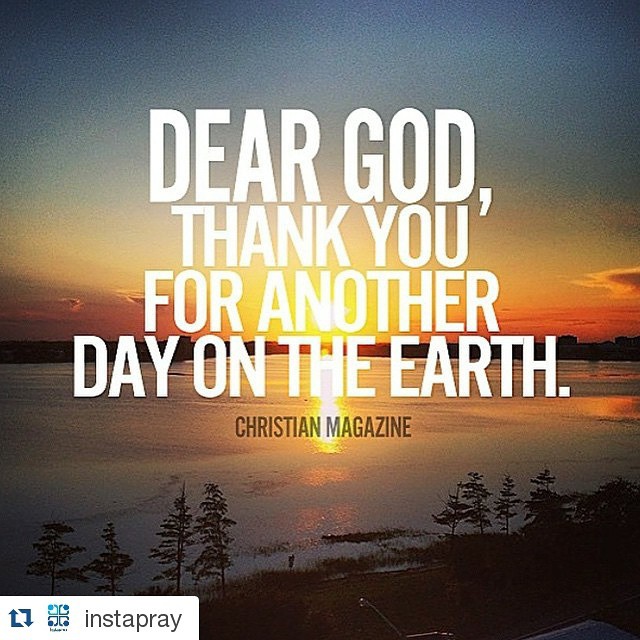The image portrays a stunning, digitally-altered sunset landscape, likely designed for a social media post by a Christian group. It features a serene lake with an orange glow cast by the setting sun. In the foreground, lush pine trees frame the scene, leading to a walkway that extends towards the water, surrounded by tall grasses. Distant mountains and scattered buildings are faintly visible against a sky transitioning from pink near the horizon to deep blue above, accented with a few clouds. Superimposed on this picturesque view, white text reads, "Dear God, thank you for another day on the earth," while black text at the bottom denotes "Christian Magazine." The bottom left corner includes a retweet icon with the label "Insta Pray," indicating its intention for sharing on platforms like Instagram or Facebook.